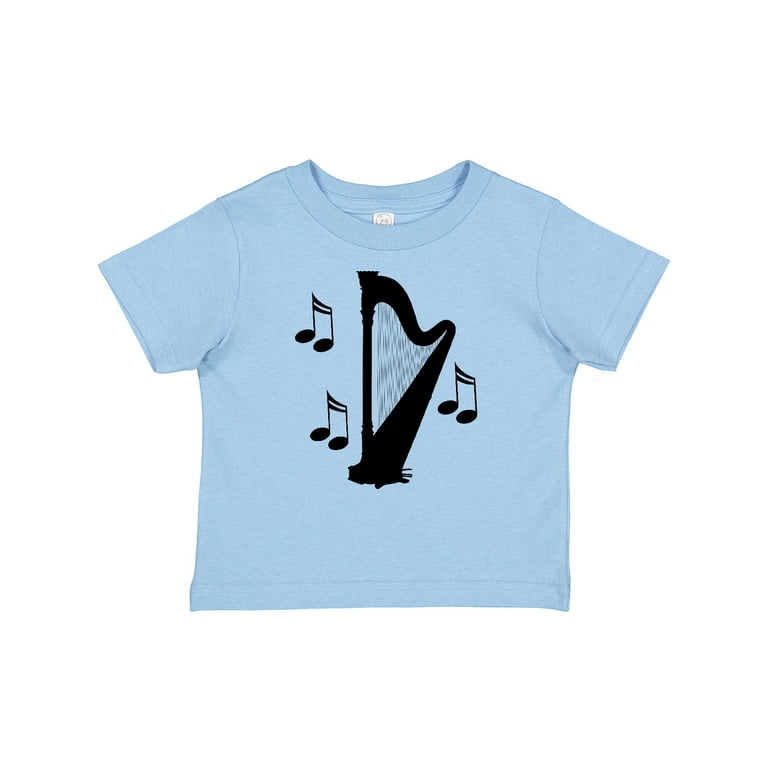The image features a light aqua blue short-sleeved t-shirt designed for children, meticulously laid out against a white background in a full-color photograph. The t-shirt has a brown collar and a crew neck, and appears slightly short in size. A large, black-outlined harp is prominently printed on the chest. Surrounding the harp are three sets of detailed musical notes: two sets on the left and one on the right. Each musical note consists of two bars at the top, with one stick and a darkened dot at the bottom. The t-shirt is neatly smoothed out with no visible ripples, and a white tag with a logo is visible inside at the back.